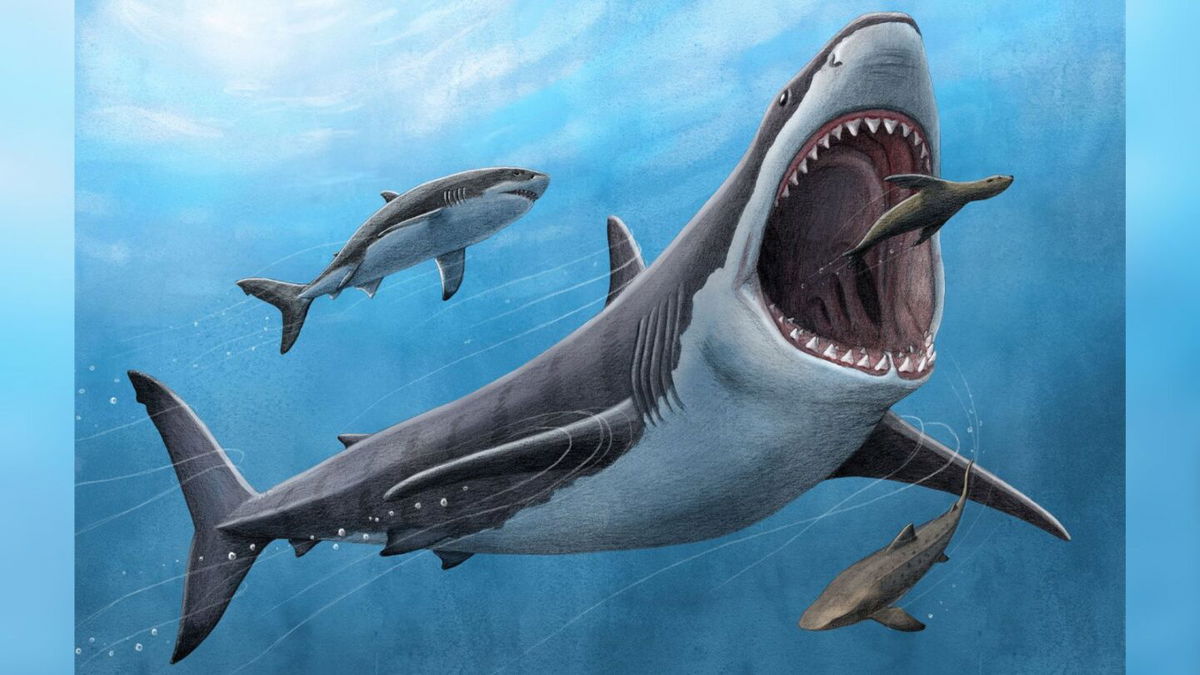The image is a highly detailed depiction, possibly a computer animation, of a dramatic ocean scene featuring three sharks and a seal. Central to the scene is a massive great white shark with its mouth gaping wide open, showcasing its sharp teeth and the textured, folded interior of its mouth. This great white is oriented downward, its formidable size dominating the image. Near its open jaws, a seal, positioned upside down, frantically swims away in a desperate attempt to escape. The water surrounding them is depicted in vibrant blue hues, interspersed with thin, white streaks of light, enhancing the dynamic underwater environment. In the background, one smaller great white shark—mouth closed and merely cruising along—swims parallel to the central shark. Another shark, possibly a remora, is located beneath the great white, moving away from the action. The intricate details and the behavior of the sea creatures contribute to the thrilling and lifelike quality of the illustration.